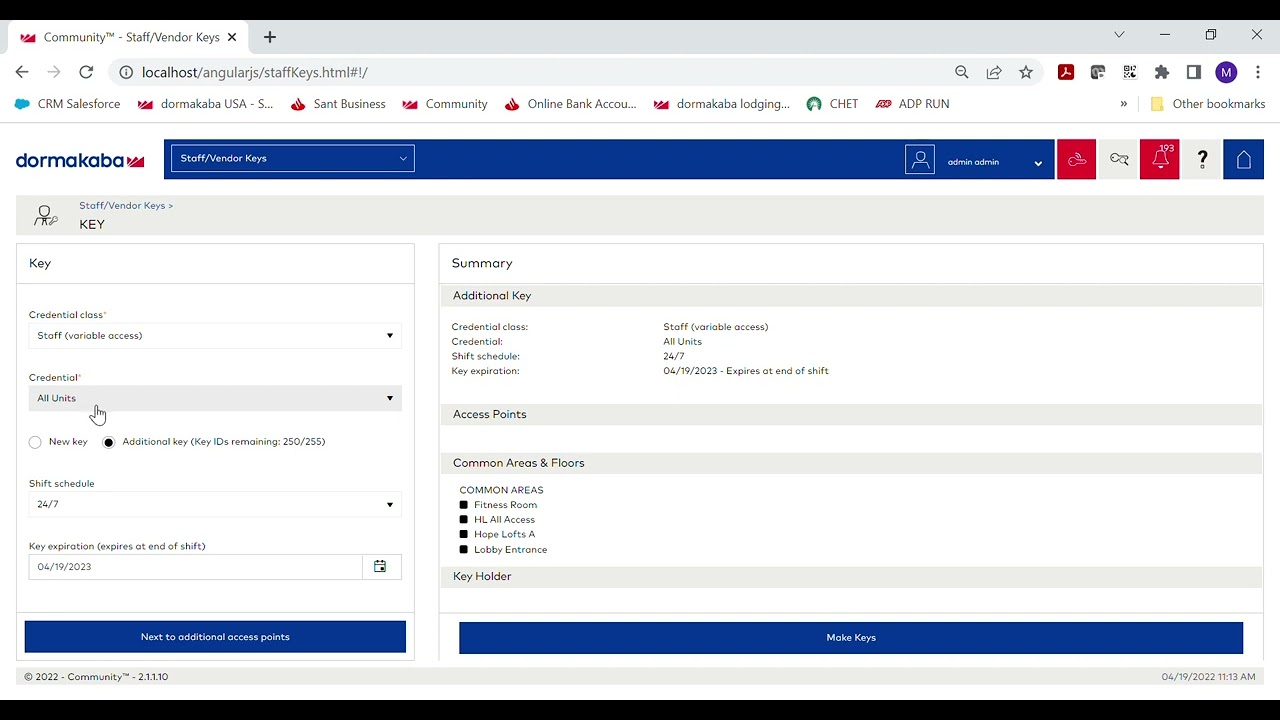This screen recording showcases an interface displaying key information for community staff and vendors. The top section is labeled "Community Staff/Vendor Keys Dorma Kaba," presented on a blue tab with a silhouette icon. Below this are columns with alternating red and white squares. 

One column is titled "Key" and contains entries such as "Staff," "All Units," "New Key," "Additional Key," and "Shifts." Adjacent to these entries, there are details about access points, with dates listed next to each. The summary section provides information on additional keys, shift schedules, and expiration at the end of shifts. It specifies access coverage for all units, common areas, floors, the fitness room, all access points, loft, and lobby entrance. There are also options for "Key Holder" and "Make Keys," likely pertaining to the creation of swipeable hotel-like keys.

At the bottom of the screen, there's a list titled "Other Bookmarks," which includes entries for "St. Bernard's Community," "Online Bank Account," and "Lodging."